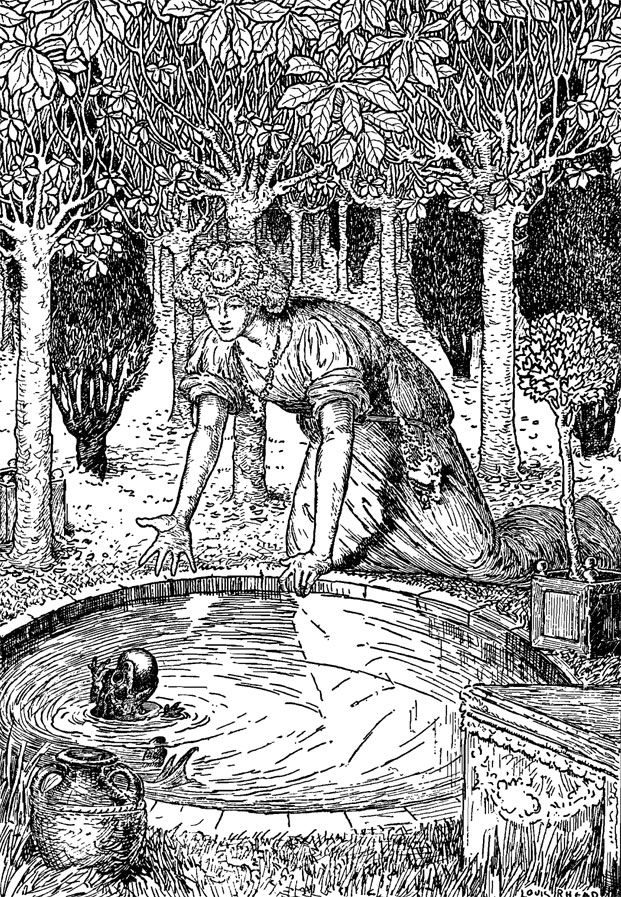This is an intricate black and white pen and ink illustration reminiscent of an old book of fables or children's stories. The scene is set in a wooded area, showcasing several finely detailed white trees with white leaves on both the left-hand and right-hand sides. In the background, a gazebo structure supported by white pillars stands among flowering trees and dark bushes.

In the focal point of the image, a woman dressed in a soft, gauzy Grecian gown is depicted by the edge of a round stone pool filled with water. Her long, curly hair cascades down to her shoulders. She kneels by the pool, her arms resting on its edge, with her right arm extended towards a small frog in the water. The frog appears to be holding or interacting with an object—perhaps an apple or ball—that the woman may have dropped or is attempting to retrieve.

In the lower left corner of the illustration, there is a finely detailed pottery pitcher, presumably used by the woman to collect water from the pool. On the right-hand side, a piece of stone suggests the form of a bench or possibly a chest, completing the picturesque and harmonious forest setting. The image is rich with shading through stippling and the use of precise lines, lending it a highly detailed and textured appearance.